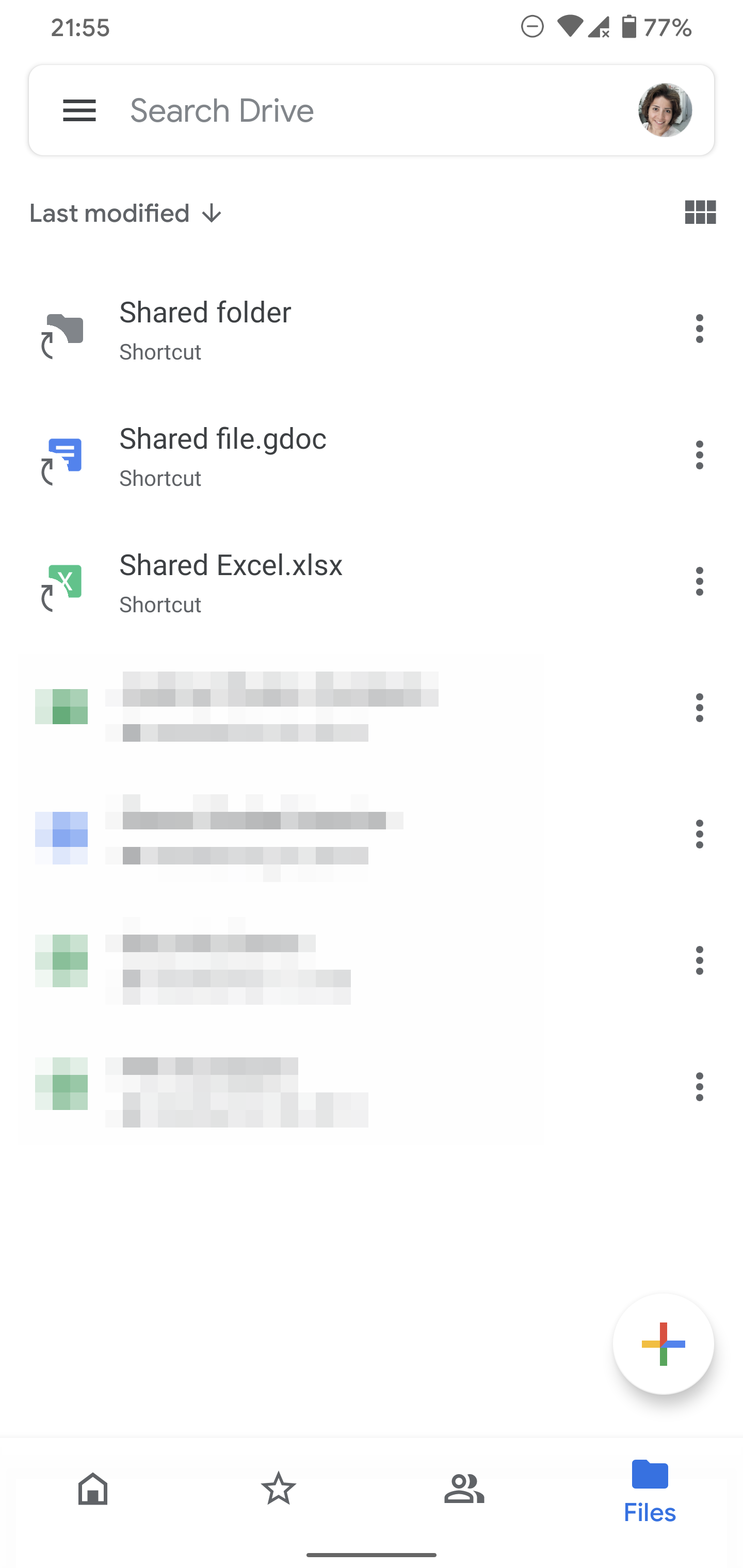A detailed view of a Google Drive interface is shown, featuring the 'Search Drive' option at the top for conveniently locating files. The account profile image, a small thumbnail of a person with chin-length brown hair, is visible, suggesting it might be a woman. Below the search bar, a list of recently modified items is displayed, including various file types such as 'shared folder shortcut,' 'shared folder file,' '.gdoc shortcut,' and 'shared Excel file.' There are indications that four additional documents are present but are redacted for privacy reasons. Each file enlisted has icons in blue or green, denoting different categories or statuses, with corresponding three-dot menus adjacent to them for further actions like editing, moving, deleting, or sharing. Additionally, a three-line menu icon next to 'Search Drive' likely provides further management options for the drive. At the bottom of the interface, four navigational icons are visible: a home icon, a star icon, a person icon, and a files icon, with the files icon highlighted in blue to indicate the current selection.